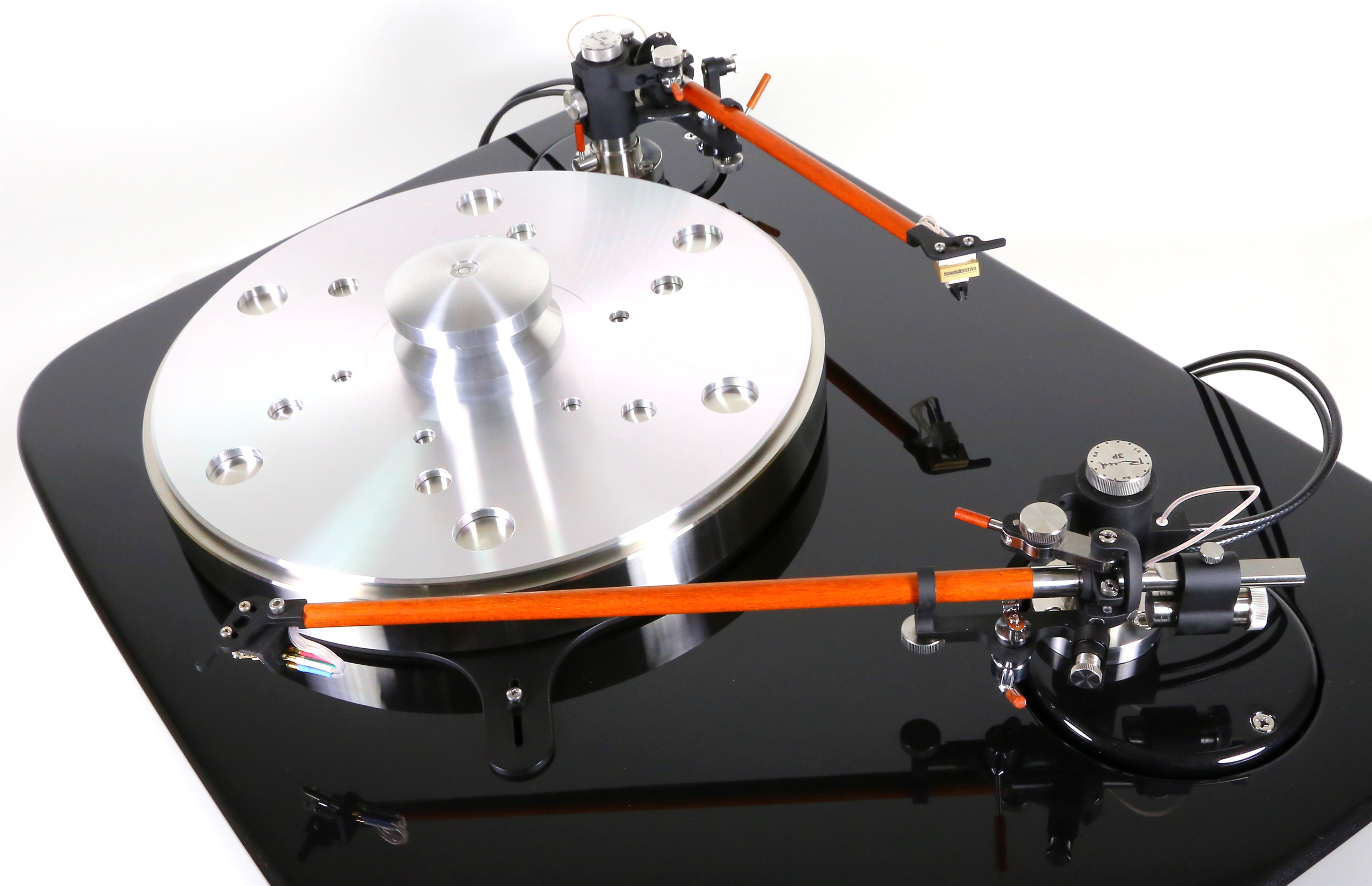The image features a sophisticated electronic media device, specifically a turntable, set against a white and light blue background. The base of the turntable is a sleek, shiny black surface that reflects the surrounding components. Dominating the setup is a bright silver circular disc situated towards the left part of the image. This disc has multiple small circular holes and a central spherical cap. Extending from the right side of the image are two needle arms, which stand out with their bright orange components. These needle arms, crucial for reading the vinyl records, feature black and silver-gray knobs and nuts and bolts, with wires attached. The remarkable detail captured includes the reflective quality of the black base, which mirrors the needle components, enhancing the overall high-tech and polished aesthetic of the turntable.